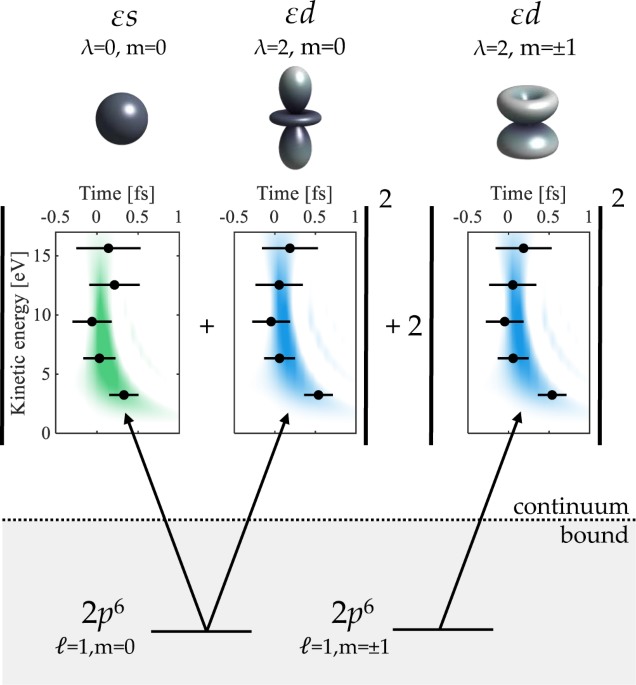This scientific poster illustrates the kinetic energy of three distinct 3D shapes: a sphere labeled "ES" on the left, a pacifier-like shape labeled "ED" in the middle, and a yo-yo-like shape also labeled "ED" on the right. The top section of the poster displays these shapes clearly. Directly beneath each shape, there are respective charts featuring lines marked with dot notation, organized vertically from 0 to 15. These charts are divided into three sections, each graph extending horizontally with labels for time progressing from -0.5 to 1.

The first chart, associated with the sphere (ES), is highlighted in green, while the charts for the pacifier-like (ED) and yo-yo-like (ED) shapes are highlighted in blue. All charts adhere to the same structural format. A continuum or bond line runs horizontally across the middle bottom of the image.

At the bottom of the poster, there are two formulas indicating energy levels: "2p^6," "e=1," "m=0" on the left and a similar formula "2p^6," "e=1," "m=1" on the right. The arrows on the dotted line point towards each shape from the bottom portion, specifying the continuum bond and linking it to the shapes' kinetic energy representations.